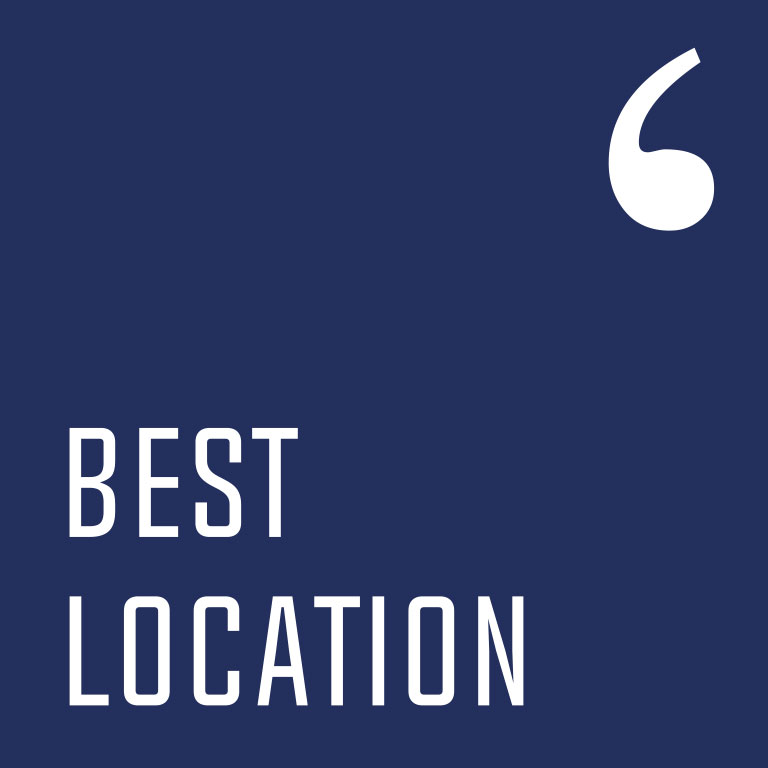An image featuring a very dark blue, square-shaped background. In the upper right corner, there's a prominent single white quotation mark. In the lower left corner, the words "BEST" and "LOCATION" are written in bold, all-caps white lettering, positioned one above the other. The text extends almost to the middle of the image horizontally.